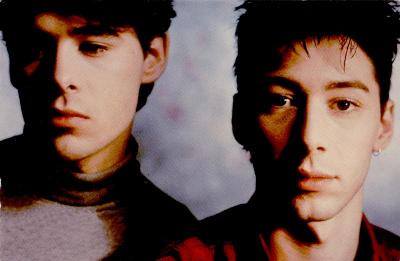In this detailed close-up image set against a blurry, grayish background, two young men in their twenties are captured with neutral expressions. On the right, a man with short, possibly piled-up black hair and a small hoop earring gazes directly into the camera. He has brown eyes and a slender nose, and wears an open red collared shirt. To the left, the other man has slightly longer, brown hair that just reaches over his ears. His eyes are cast downward, giving him a downcast appearance, with lips turned downward at the corners. He wears a grayish turtleneck. Both men share bushy eyebrows and strikingly similar facial features that suggest they might be related or part of a duo, possibly in a music group. The bright lighting highlights their identical brown eye color and the similar texture of their skin. Overall, the image conveys a sense of reserved, yet intense, presence from both individuals.